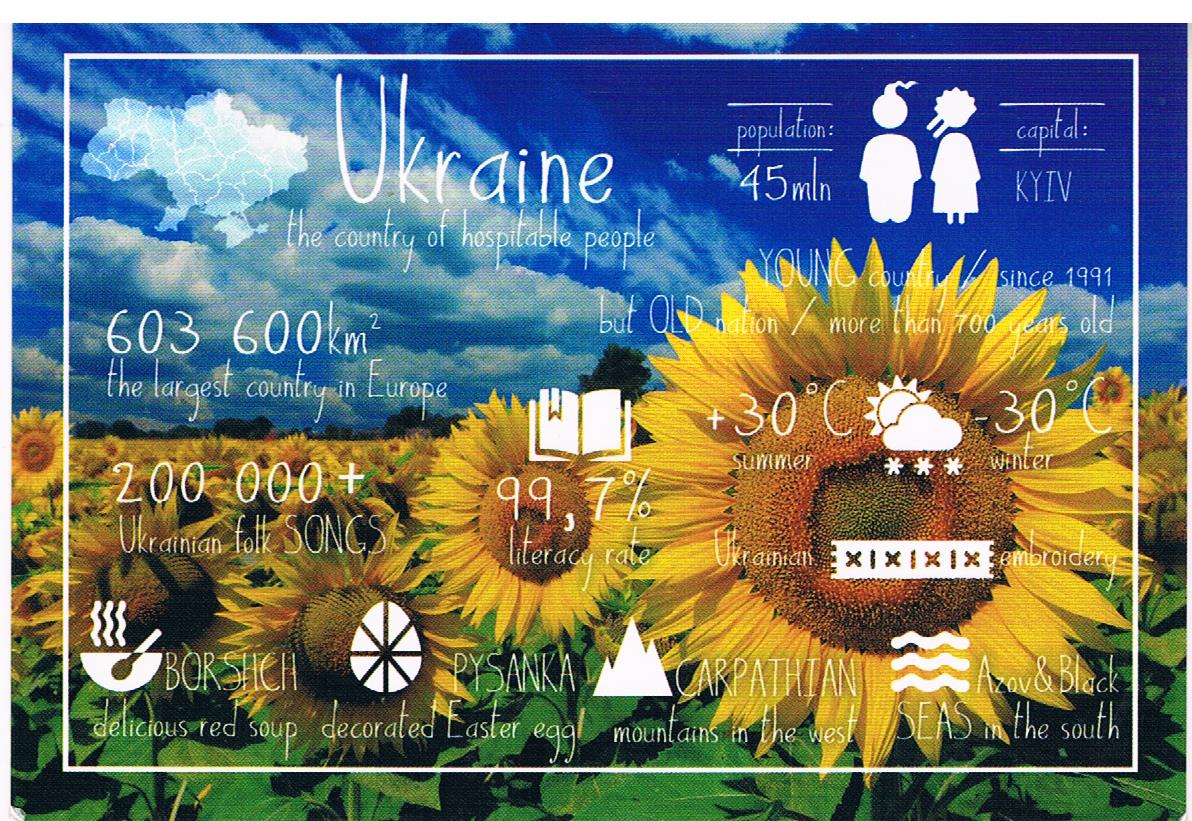This vibrant and detailed image, resembling a promotional poster or postcard for Ukraine, showcases a picturesque outdoor scene under a clear blue sky with white and gray clouds. Central to the image is a vast, colorful field of large, radiant sunflowers with green leaves, stretching towards the horizon where distant trees are visible. The poster features rich colors, including shades of blue, white, gray, yellow, orange, and green, accentuating the natural beauty of the landscape. 

Prominently displayed text provides insightful information about Ukraine: "Ukraine, the country of hospitable people, population 45 million, capital Kiev. Spanning 603,600 square kilometers, it is the largest country in Europe. A young country since 1991, but an old nation with a history of more than 700 years. Home to over 200,000 Ukrainian folk songs, a 99.7% literacy rate, summer highs of +30°C and winter lows of -30°C. Renowned for its Ukrainian embroidery, borscht (a delicious red soup), decorated Easter eggs (pysanka), the Carpathian Mountains in the west, and the Azov and Black Seas in the south." 

Overall, the poster effectively highlights Ukraine's natural beauty, rich cultural heritage, and significant historical background.